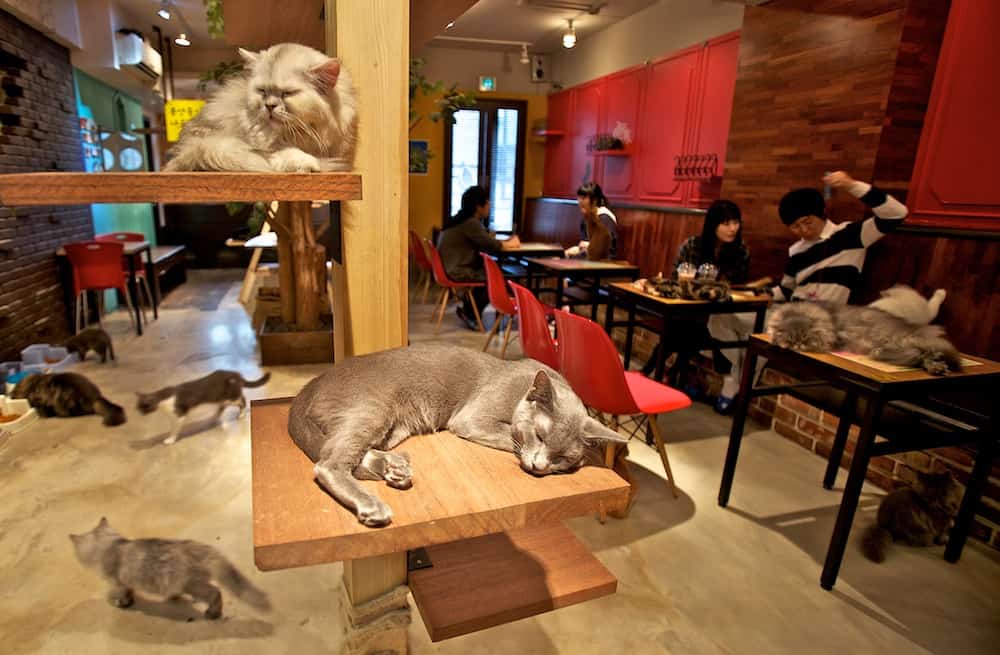The image captures the vibrant scene of a bustling cat cafe in Japan. The cafe's interior blends a mix of exposed brick and various materials, with a warm and inviting ambiance. A central feature is the extensive cat jungle gym made of wood, featuring platforms both on the ground and elevated on tables. Cats, in a spectrum of colors including black, white, gray, orange, red, yellow, and green, can be seen lounging, playing, and even napping on these wooden structures. 

Front and center, a gray cat naps on a wooden square, adding to the cozy atmosphere. The cafe is furnished with small square tables with black legs, surrounded by bucket seats in various shades of red and chairs made of light brown wood. A long wooden bench with reddish-brown planks and a red brick wall underneath spans one side of the cafe, bordered by shelves holding cat trees and other decorations. The walls are diverse in color: red panels above the bench, yellow in the back, and a teal hue on the left, all beneath a white-painted ceiling.

Several patrons enjoy their bubble tea and other refreshments at these tables, including two couples in the background—one sporting black and white attire, the other in cozy sweaters. Cat cafes, popular in Japan and gaining traction in America, offer a unique experience where visitors can relax with drinks and snacks while interacting with the resident cats, and sometimes even adopt them.